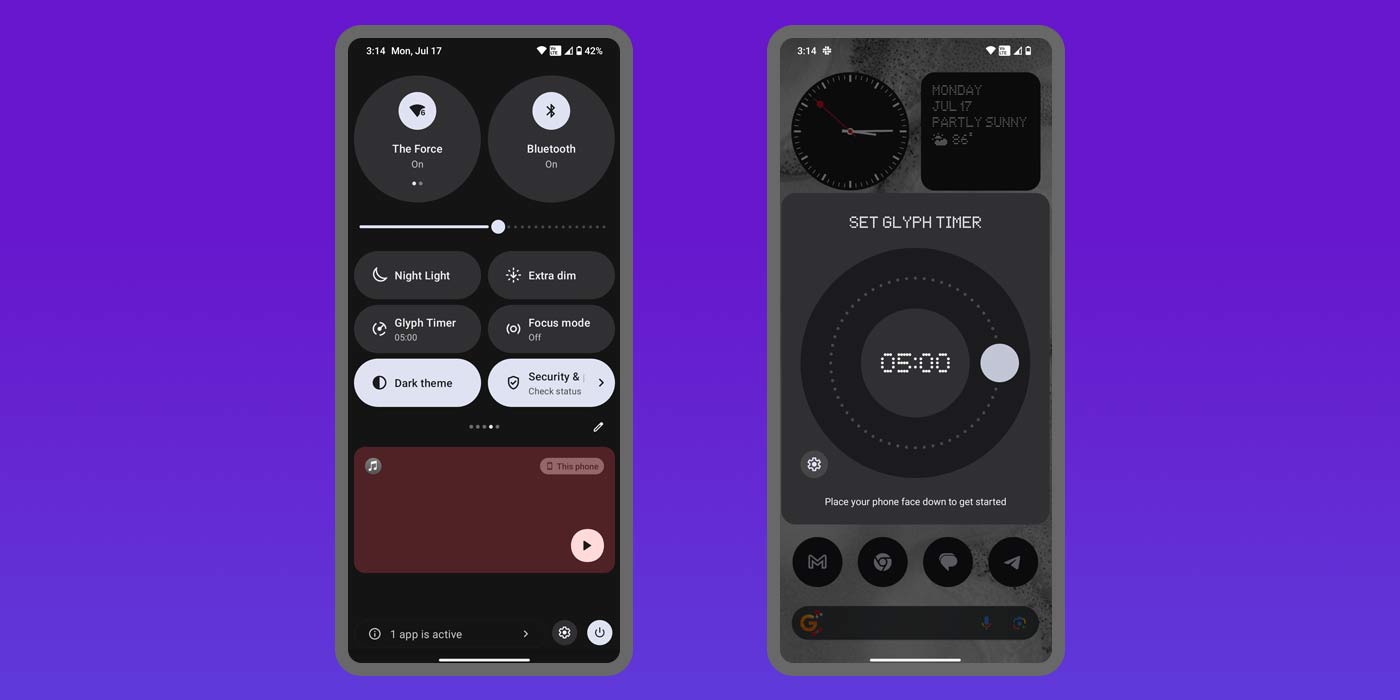This image features a medium purple background, against which two smartphones are displayed side by side. Both smartphones have medium gray borders. The smartphone on the left has two dark gray circles positioned side by side near the top. Within each of these dark gray circles are two smaller white circles, each containing an icon, with text underneath that is too small to readable. The right phone appears to display "Bluetooth" text in a similar position.

Below these icons is a status bar, followed by a row of six buttons. The labels on the buttons are challenging to decipher but seemingly read "Night Light," "Extra Sun," "Glyph Timer," "Dark Home," and two other text elements that are indistinct. Below these buttons is a burgundy box.

The smartphone on the right has a dark gray box towards its center, containing a circle with the inscription "05:00."